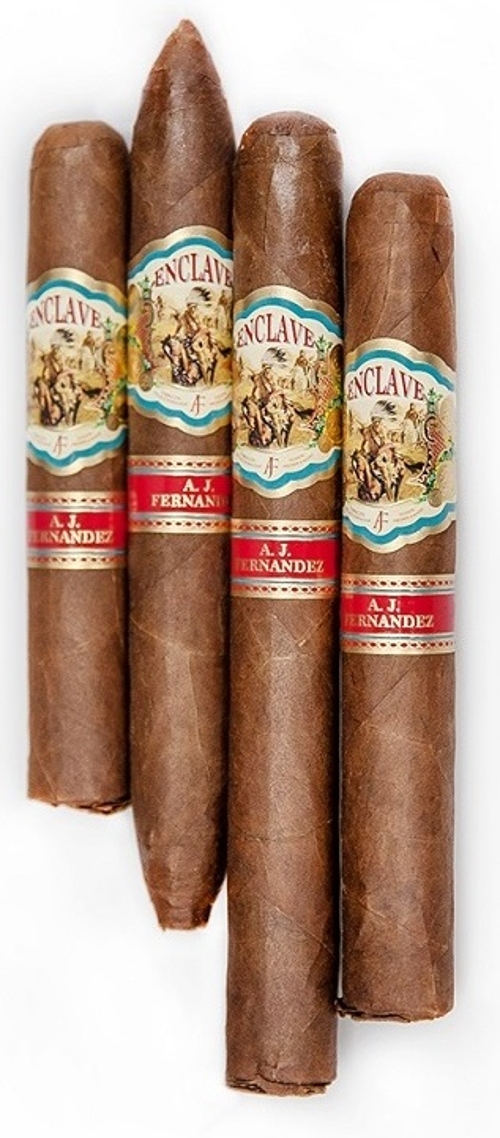The image depicts four cigars of varying lengths and shapes arranged vertically next to each other. Each cigar features a label that reads "Enclave" with a blue border. The label also contains a detailed golden illustration of an Indian chief riding a horse, adorned with a headdress. Beneath this, there is a red band with the name "A.J. Fernandez" written in gold uppercase letters, flanked by two golden strips. One of the cigars is torpedo-shaped with a taper at both ends, while the others vary in length but are flat at one end and slightly tapered at the other. The cigars appear robust and well-crafted, likely suggesting a premium and possibly expensive product.